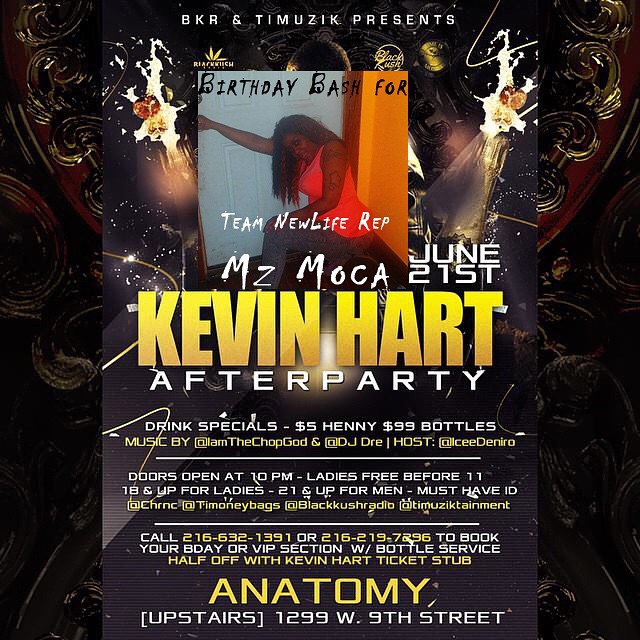The image showcases a vibrant poster set against a dark, intricately designed background. Dominating the top portion, in bold white letters, it reads "BKR and Timusic Presents." Just below this, it announces "Birthday Bash for Team New Life Rep, MZ Mocha," accompanied by a photo of a woman with long black hair in an orange top, sitting on a stoop and looking to the left.

Central to the poster, in striking yellow letters, the name "Kevin Hart" is prominently displayed, indicating he is the star attraction. Following this, "After Party" is declared in white letters. 

The poster further details enticing drink specials like "$5 Henny" and "$99 bottles." It notes that doors will open at 10 p.m., with free entry for ladies before 11 p.m., and specifies age requirements—18 and up for ladies, 21 and up for men, with ID required. 

Additionally, music is provided by at Lamb the Chop God and DJ Dre, with hosting by C De Niro. For those looking to book a VIP birthday section, a contact number is provided.

At the bottom, "Anatomy Upstairs" is boldly written in large yellow letters, with the venue's address, "1299 West 9th Street," listed directly below.